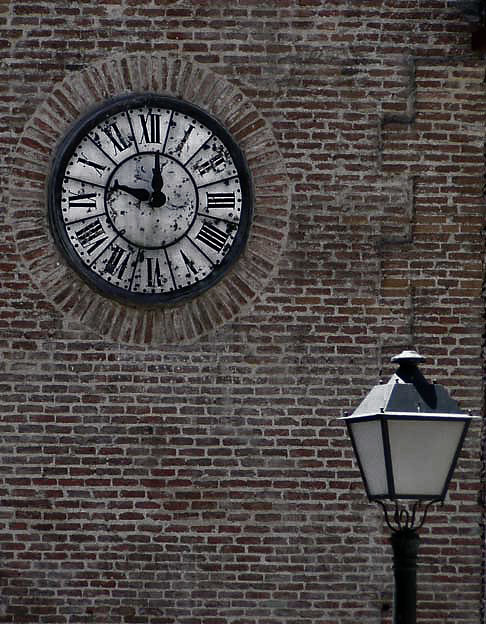Captured in bright daylight, this detailed photograph showcases a red brick building with prominent light-colored cement grout. Dominating the upper left portion of the image is a large, open-faced clock with distinctive Roman numerals and decorative black hands, pointing somewhere between 9 and 10 o'clock. This clock is encircled by an intricate brick pattern, adding to its significance against the dark brick façade. In the lower right-hand corner, a black street lamp emerges, topped with a metal point and four clear protective shields around its white glass bulb. The scene is bathed in sunlight, highlighting the textures and details of the building and the street lamp.